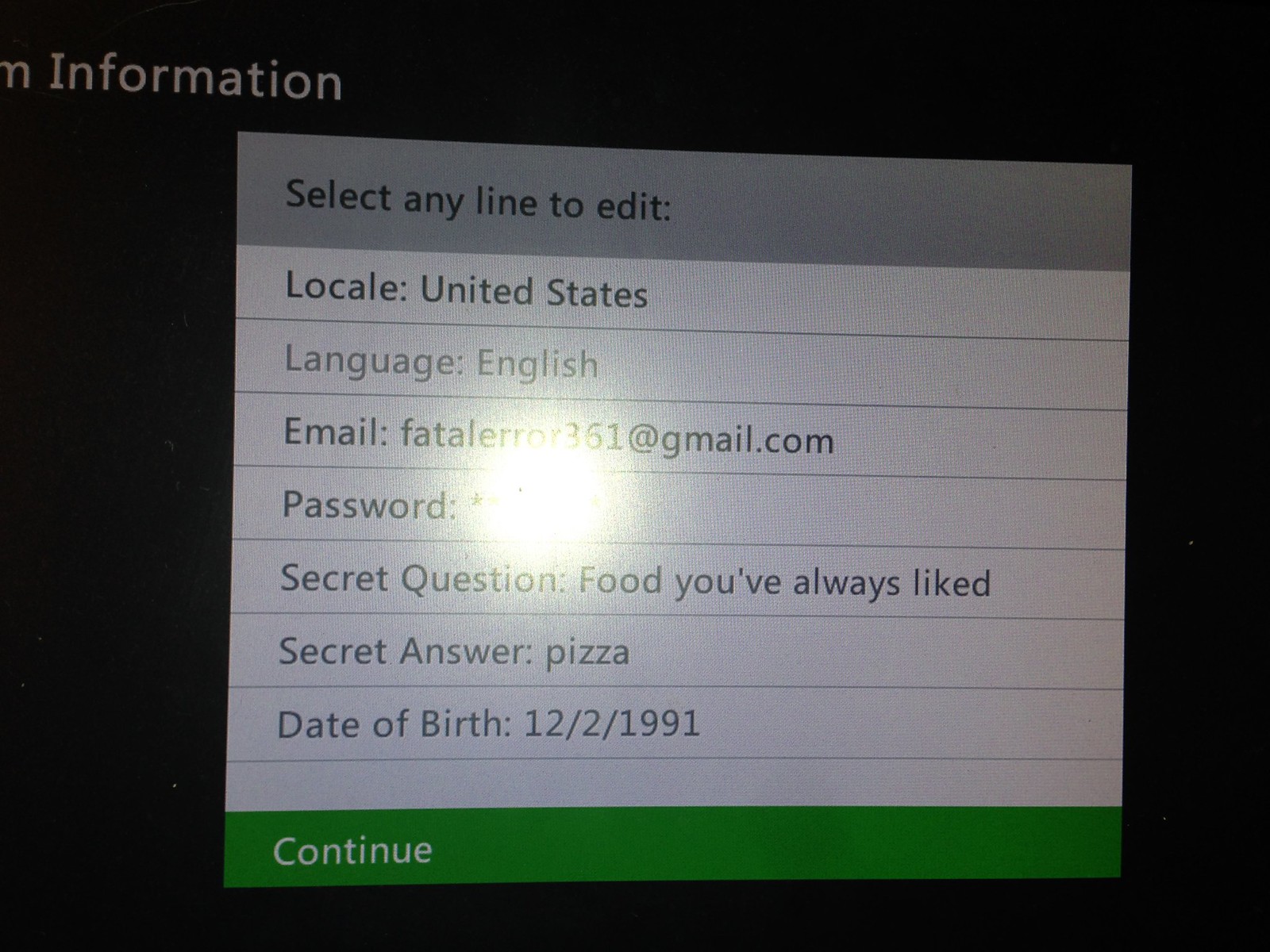The image depicts a computer screen with a black background and a prominent white box in the center, containing editable fields. At the top of the box, the heading "Information" is visible. Below it, instructions read "Select any line to edit." The fields listed are as follows: "Locale: United States," "Language: English," "Email: fataleerror361@gmail.com," followed by a partially obscured "Password" field due to a bright flash from the camera. Further down, it includes "Secret Question: Food you’ve always liked," with "Secret Answer: Pizza," and "Date of Birth: 12-2-1991." At the bottom of the box, a green bar with the text "Continue" suggests the next step in the registration process.